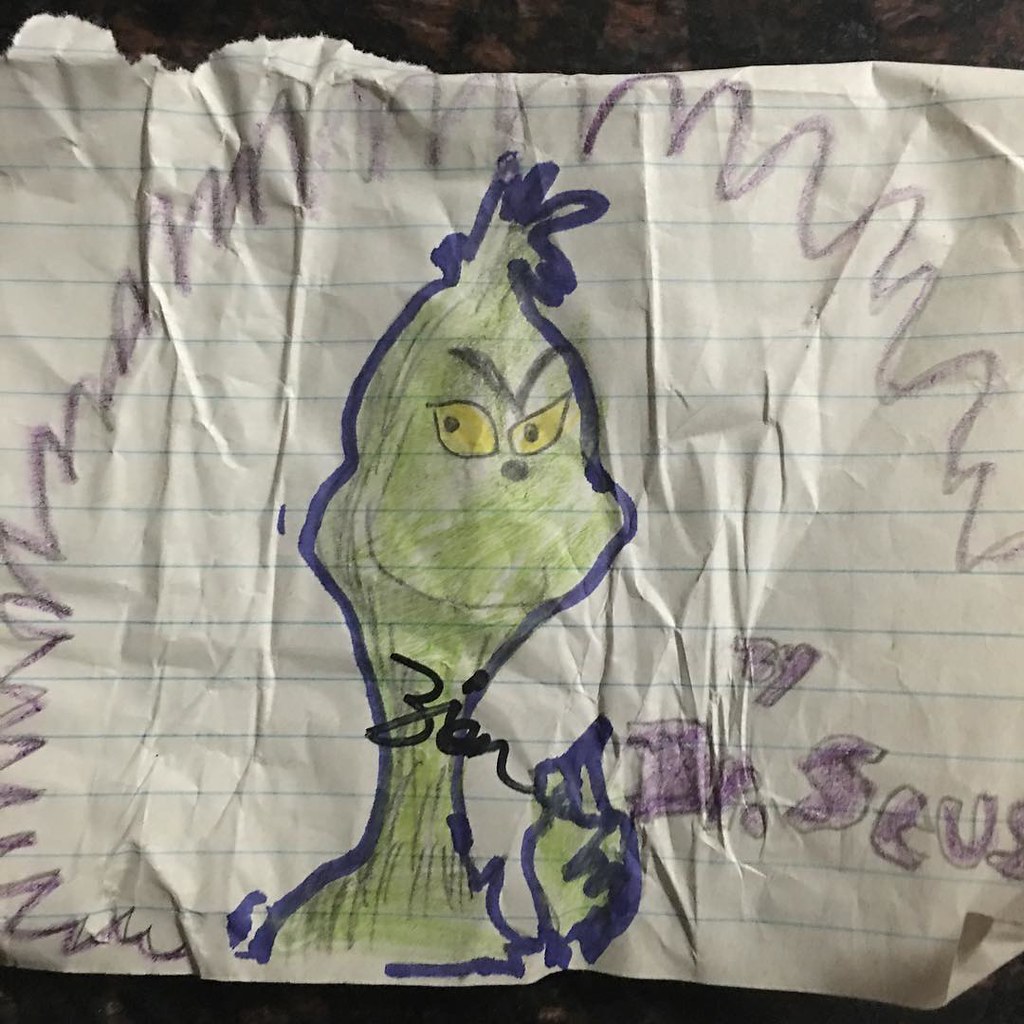This is a photograph of a piece of notebook paper that appears to have been torn out of a notebook. The paper is slightly wrinkled and has a folded up bottom right corner, suggesting it has been handled or wadded up. The central focus of the drawing is the Grinch, a character created by Dr. Seuss, sketched in a mixture of pencils, markers, and crayons. The Grinch is depicted from his shoulders up, outlined in blue marker with scraggly details emphasizing his green fur. His filling is colored with a lighter green, likely crayon or marker, and he displays his signature mischievous frown and yellow eyes, looking off to the side. Above his head is a small tuft of fur, while a jagged, burst-like outline surrounds him, drawn in purple marker. To the right of the drawing, in bubble-like purple lettering, it reads "by Dr. Seuss", partially obscured but still legible. Near the neck of the Grinch, the name "Ben" is written. The detail and recognizable features, despite the rudimentary style, suggest this drawing was created by a child.